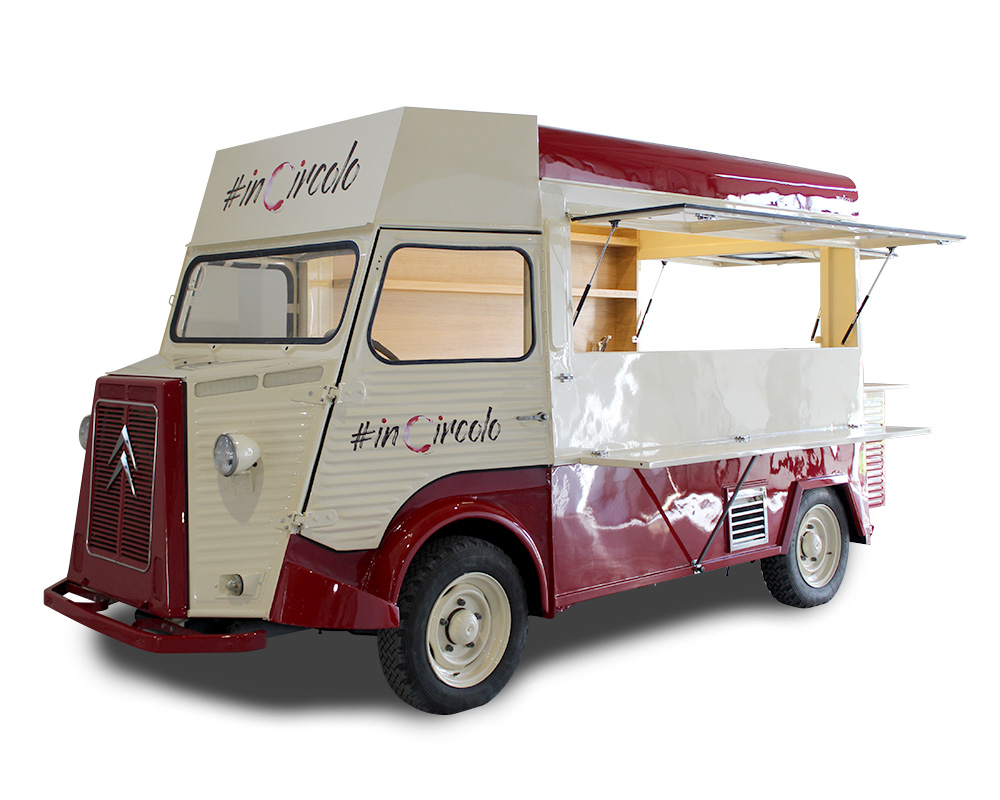The image features a meticulously detailed, restored vintage food truck or vendor truck, possibly a computer-generated image due to its lifelike appearance. The vehicle sits against a white background with a Photoshopped drop shadow, further emphasizing its isolated presence in the image. The truck's exterior displays a glossy dark red color spanning the entire length of the vehicle, except for the hood and top of the windshield, which are white. The grill also features red with chrome accents, and the front bumper is red. Above the windshield, handwritten in black, is the hashtag "#incircolo," with a distinctive 'C' resembling a red and white coffee stain ring.

The driver's side door, or the left front door, bears the same "#incircolo" logo. The tires are black with white wheels. A unique feature of the truck is the hydraulically supported top half of the side wall that opens to reveal the brown interior, which includes wooden shelving against the far left wall and a folding white bench supported by a little black bar. There is also a small shelf below the opening, typical of food trucks for serving customers. The back roof of the truck is colored red. Overall, the image portrays a pristine vintage food truck with meticulous detailing.